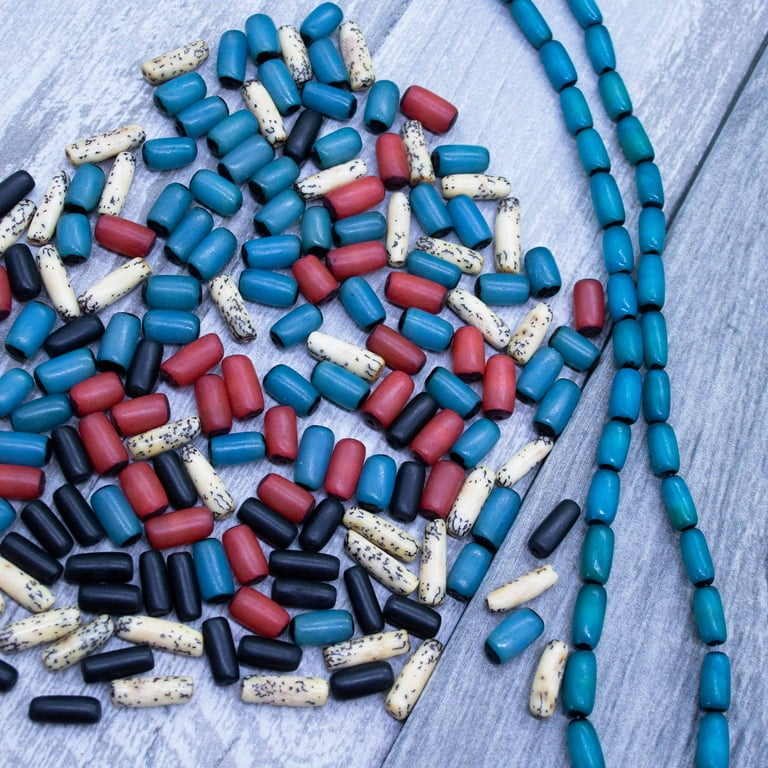The square-shaped photograph, approximately six inches by six inches, features a background of diagonally arranged wooden planks, stained or painted in various shades of blue. The majority of the left-hand side of the image is occupied by an array of loose, long cylindrical beads in blue, red, black, and white with black specks, which appear to be natural stone or gemstone beads. On the right-hand side, two strands of blue cylindrical beads, forming a necklace, extend from the top and run off the bottom of the frame, with a slight shine visible on the beads. These strands and scattered beads sit upon the blue-toned wooden planks, creating a visually appealing contrast. The source of lighting in the photograph is ambiguous, making it unclear whether the image is taken indoors or outdoors.